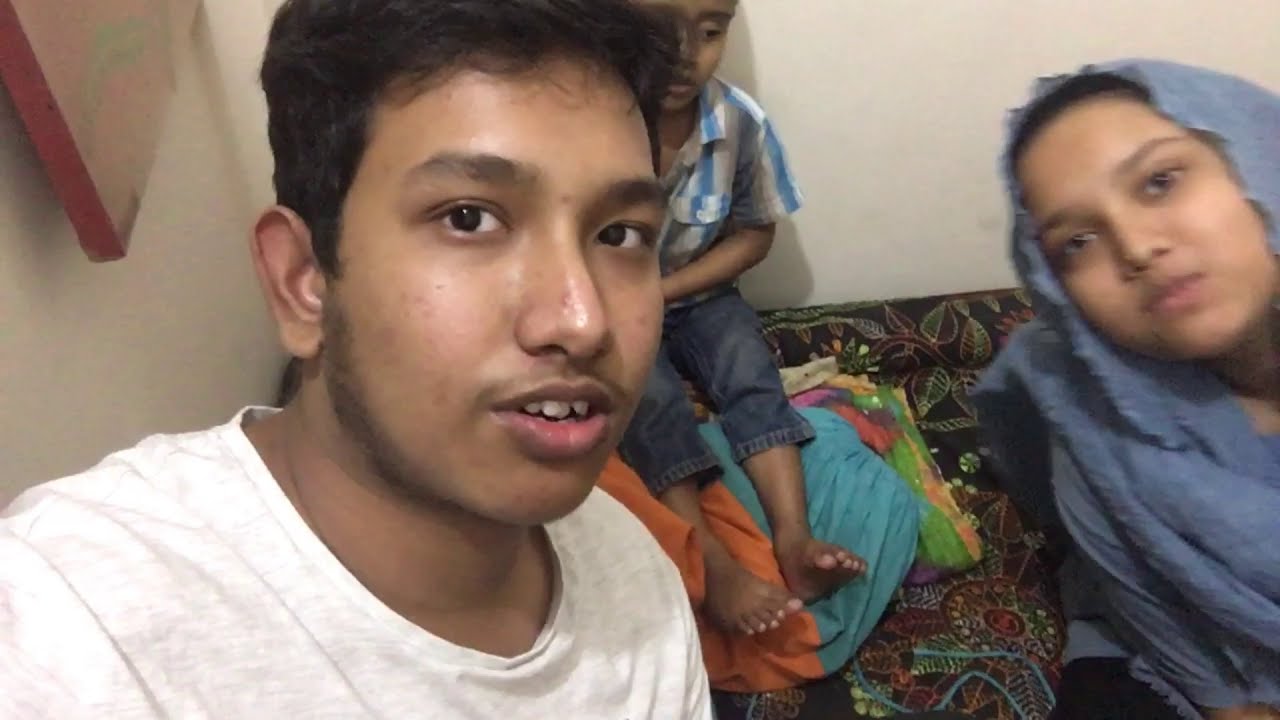This image is a selfie of three people in a room with a black, multi-colored leaf-patterned couch and a geometric-pattern section. On the left, partially visible in the foreground, is a man in a white t-shirt with short dark brown hair and caramel-colored skin, likely South Asian. He has a minor blemish on his nose and a bit of facial hair. Behind him and to his right sits a little boy wearing a vertically striped blue, gray, and white collared shirt, dark blue jeans that look like shorts, and bare feet. The boy is seated on the couch, and beneath his feet are some scattered clothes in purple, blue, and green hues. Further to the right is a woman wearing a light blue sari covering her head, implying she is also of South Asian descent. Her black pants are partially visible. The room has a white wall with a portrait or painting hanging behind the man in the white shirt.